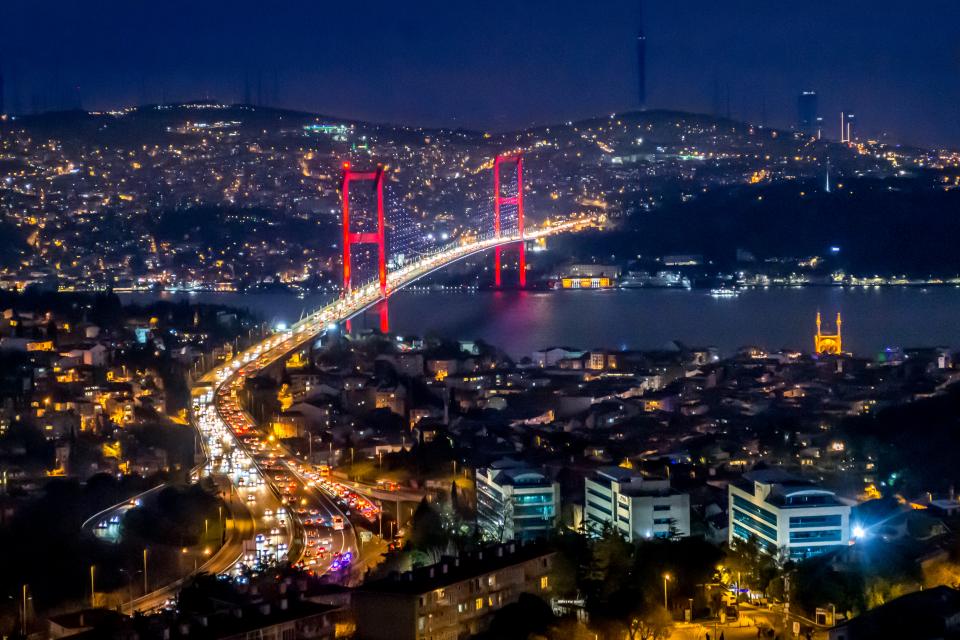This is a detailed photograph of a bustling cityscape at night featuring a river that runs horizontally along the middle ground. On either side of the river, the city is ablaze with the lights of hundreds of homes and businesses, extending into the background where a hilly mountain silhouette punctuated by a few radio towers subtly frames the scene. The skyline above is dark, contrasting beautifully with the city's vivid illumination. The image prominently features a brilliantly lit bridge crossing the river, its span supported by two striking red structures. The bridge, reminiscent of the Golden Gate but not exactly it, is alive with the white headlights and red taillights of countless cars in transit. In the foreground, particularly noticeable in the bottom right quadrant, are three large and modern office buildings with stylish glass windows, towering over the lit roadway where traffic flows steadily into the city. Additionally, a boat is visible on the river, adding to the dynamic nature of this vibrant nocturnal scene. Despite the initial misrecognition, the city remains unidentified but undeniably captivating.